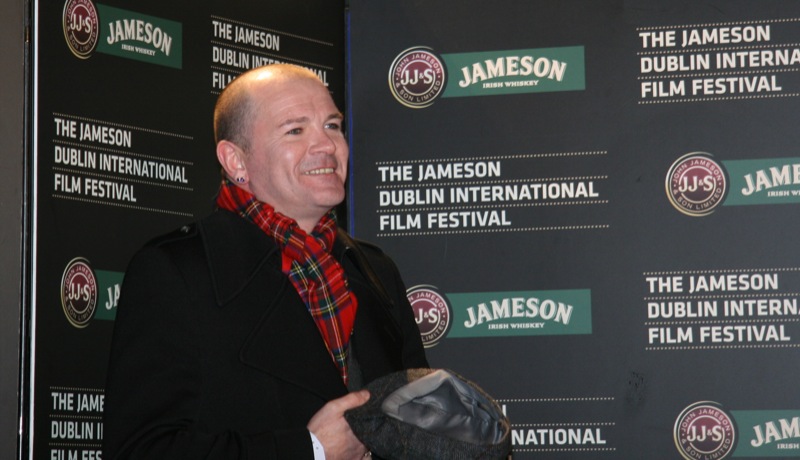The image is a rectangular photograph depicting a middle-aged white man standing slightly sideways, smiling as he looks into the distance. He has very short, almost bald hair with gray and black specks, and is adorned with earrings and eyeliner. He is dressed in a black wool overcoat over a white shirt, with a red, green, and blue plaid scarf tied around his neck and tucked into his coat. In his hands, he holds a gray hat. The backdrop behind him features the Jameson Irish Whiskey logo and the text "Jameson Dublin International Film Festival" repeated multiple times on a dark green background, indicating that the photograph was likely taken at a publicity event sponsored by Jameson Irish Whiskey. The man's appearance and the setting suggest he might be an actor attending the film festival, captured by the media.